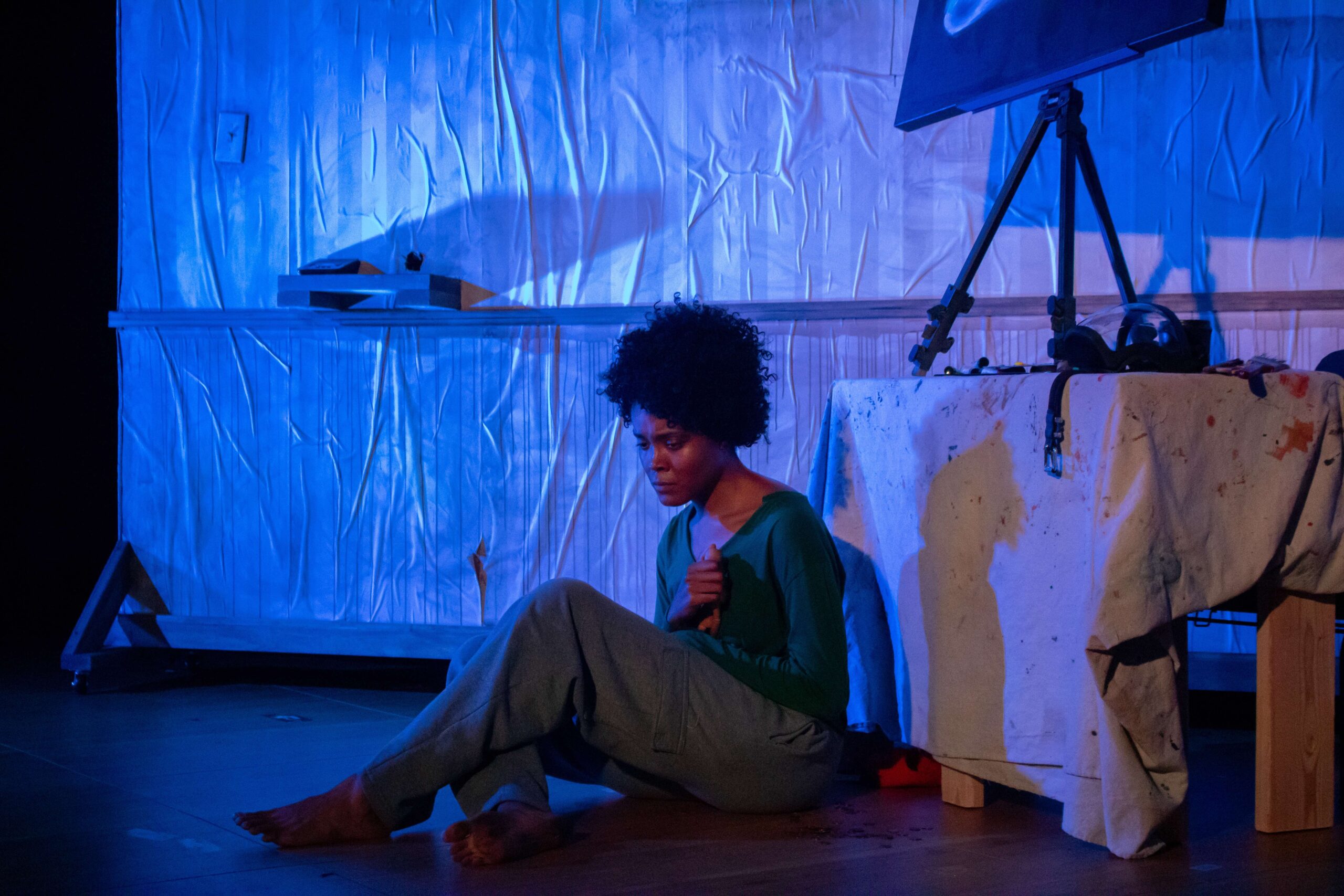In a dimly lit room that resembles an art or photography studio, a woman sits on the floor, her feet crossed and her arms resting in her lap. She wears gray sweatpants and a green shirt, and her afro-style hair frames a face marked by sadness and disappointment. The setting is shadowy, with a white wall behind her that appears to be covered in plastic or perhaps serves as a stage prop, given it is on wheels and features a light switch. To her left, a table draped in a paint-splattered white cloth holds various pieces of electronic equipment and a tripod supporting a dark-framed picture with a hint of a white semicircle. A faint beam of light creeps through the otherwise dark room, casting shadows that add to the melancholic atmosphere. The scene tells the story of a moment steeped in sorrow and introspection amid the artistic or staged surroundings.